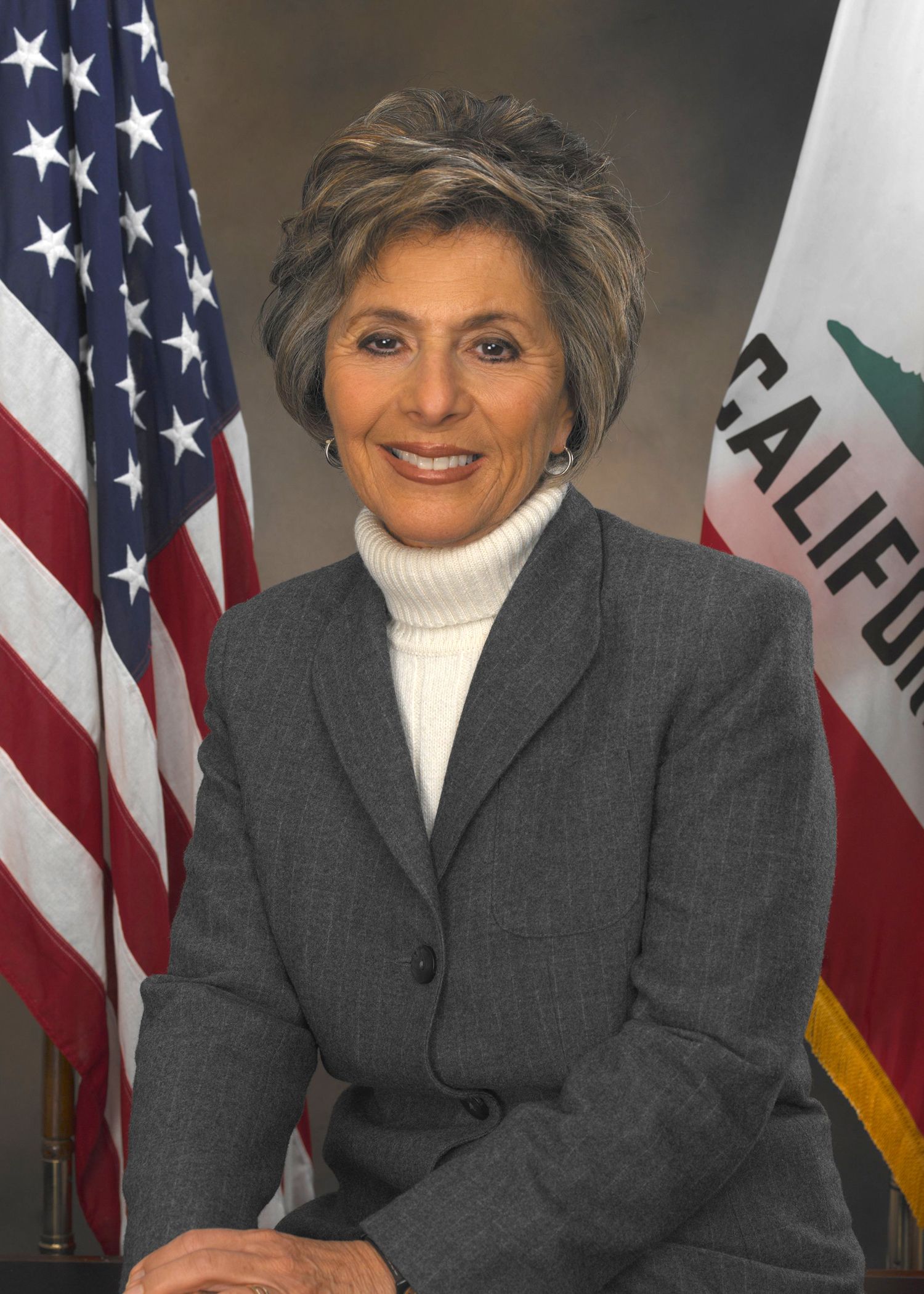The photograph features a close-up, portrait mode image of an elderly white woman who appears to be a politician. She is seated and visible from the chest up. She has well-kept, grey-white hair with hints of brown, styled in short curls that almost resemble a wig. Her brown eyes are accentuated with eyeliner and she is wearing noticeable face makeup, including lipstick. Delicately smiling and showing her top teeth, she adorns silver hoop earrings. Her outfit consists of a white turtleneck sweater underneath a buttoned grey blazer with large buttons. Behind her, an American flag is positioned to her left, displaying the familiar blue corner with white stars and red and white stripes. To her right is a partially visible white flag featuring red and yellow sections, with partially obscured text that includes the word “California.” The rest of the background is light green, enhancing the subject's prominence in the frame.